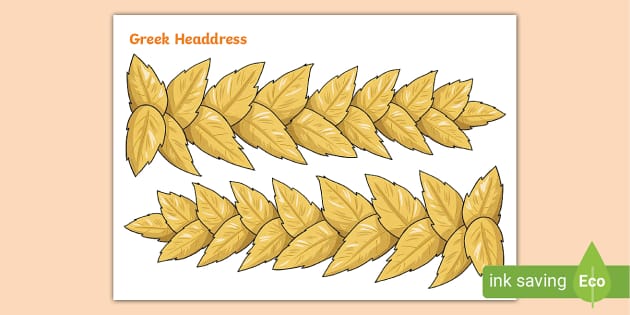This is a computer-generated illustration featuring a light beige background with a prominent coral pink rectangle in the center. Inside this pink rectangle lies a horizontally aligned white rectangular area displaying a detailed arrangement of golden yellow leaves. The leaves are organized into two horizontal sets: the upper set has individual pairs of leaves for ten rows, with the last leaf pointing right, while the lower set mirrors this pattern, ending with a single leaf pointing left. Each leaf has a delicate light gray vein running through its middle. Near the upper left corner of the white rectangle, the text "Greek headdress and brown prince" is written in orange letters. In the lower right corner, a light green rectangle bears white text reading "Ink Saving" next to a depiction of a green leaf emblazoned with the word "Eco" in white print.